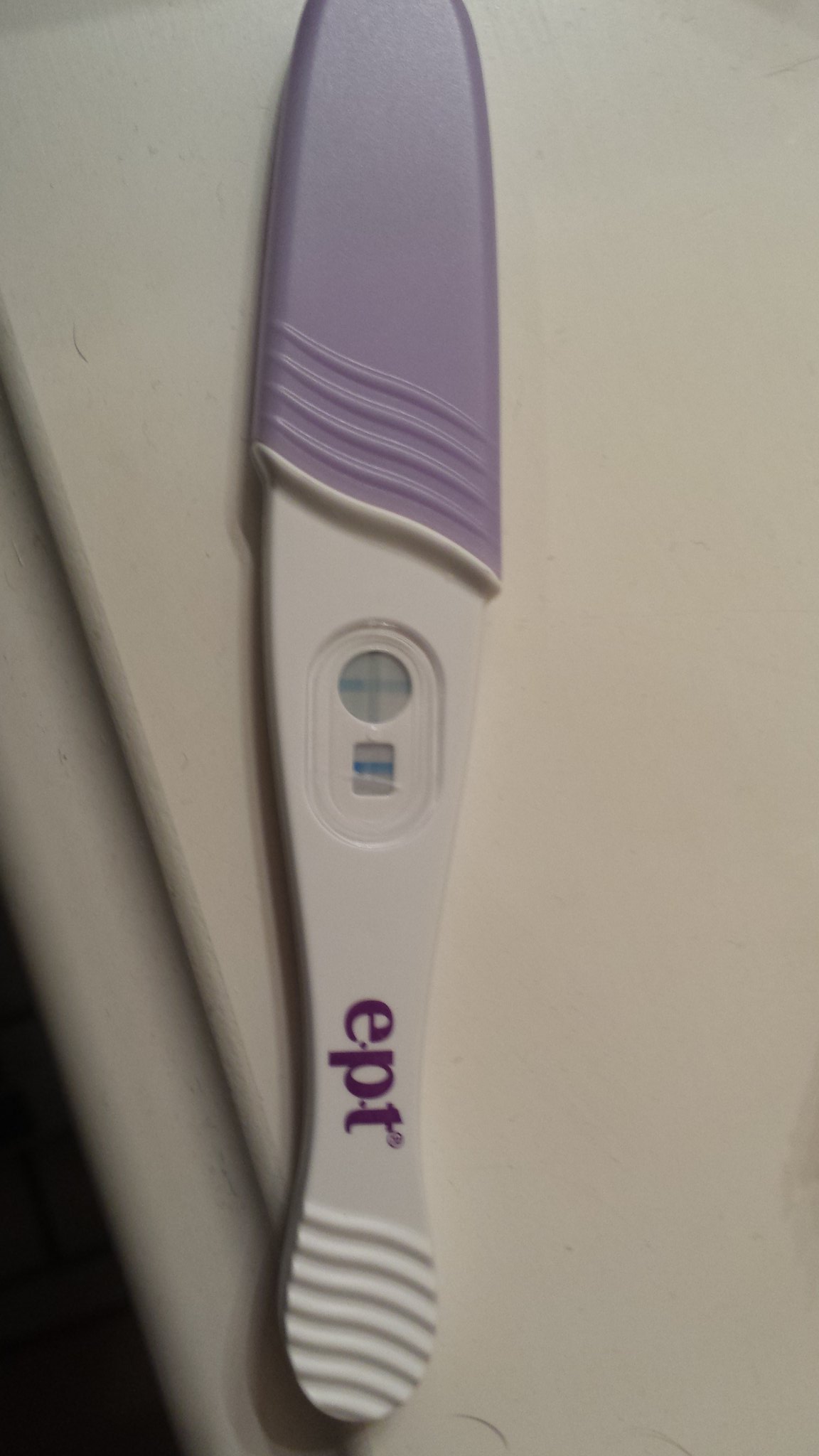The photograph features a vertically aligned plastic pregnancy test resting on the edge of a white countertop, which dominates the background of the image. This countertop, slightly rounded at the edges, fills the majority of the vertically rectangular frame, with a small triangular section of black in the lower left corner representing the floor beneath. The pregnancy test, showcasing a design divided into a white bottom half and a light purple top half, exhibits subtle diagonal raised texture lines for grip purposes. These grips are positioned at the very bottom and just above the color transition point. The test itself has rounded tips and gently curved edges, creating a smooth yet not perfectly straight outline.

The brand name "e.p.t." is printed in lowercase letters on the lower white section of the test, accompanied by a small circular logo likely indicating a trademark or registration, though the fine details inside the circle are indiscernible. The test's center displays two distinct shapes: a circular light gray window at the top housing a blue plus sign, and a square light gray window below it featuring a blue minus sign. The minus sign is rendered in a slightly darker shade of blue compared to the plus sign, adding contrast to the test’s readout indicators.